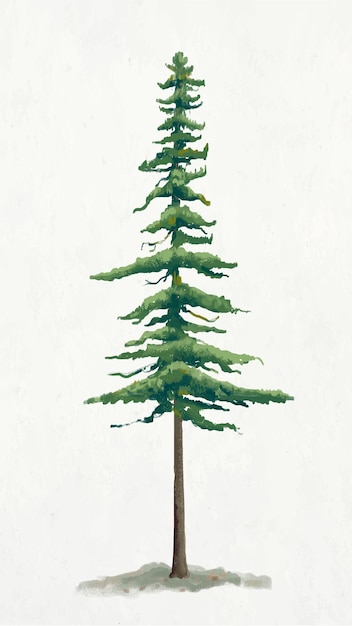This is a vertically rectangular painting set against a very faint off-white background. At its base, you can see a touch of gray representing the ground. The focal point of the piece is a tall and thin scraggly pine tree that extends upward. The trunk is relatively bare for the first half, with branches only starting to sprout about halfway up. These branches alternate between shorter and longer lengths initially, but become very short and sparse towards the top. The tree, reminiscent of an evergreen or Christmas tree but much thinner and sparser, evokes the image of a Charlie Brown tree. The painting appears to be either a cartoon visual animation or possibly a watercolor, though it remains unsigned. Overall, the scene is stark, with the solitary tree standing in the middle of an otherwise empty and monochromatic background, highlighting its frail yet resolute presence.